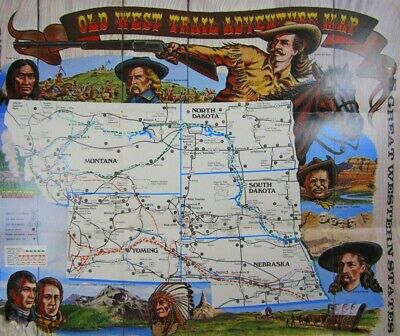The image features a mid-20th-century pen and ink illustration of a "Great Western States Trail Adventure Map," prominently showcasing a detailed map of the American West, specifically the states of Montana, North Dakota, South Dakota, Nebraska, and Wyoming. The map occupies the central portion of the poster, set against a gray, wood-panel-like background. Surrounding the map are various historical and iconic figures from the American Old West, including Teddy Roosevelt, George Custer, Crazy Horse, and presumably Lewis and Clark in the lower left corner. The poster also illustrates scenes characteristic of the Old West, such as cowboys in pioneer outfits with wide-brimmed hats, riding horses, and holding guns, as well as depictions of mountains, rivers, and caravans. At the top, a dark brown ribbon banner displays the text "Old West Trail Adventure Map" in a frontier-style font, with yellow and red block text. Additionally, the poster includes a view of a hill against a blue sky, amplifying the nostalgic feel of the illustration.